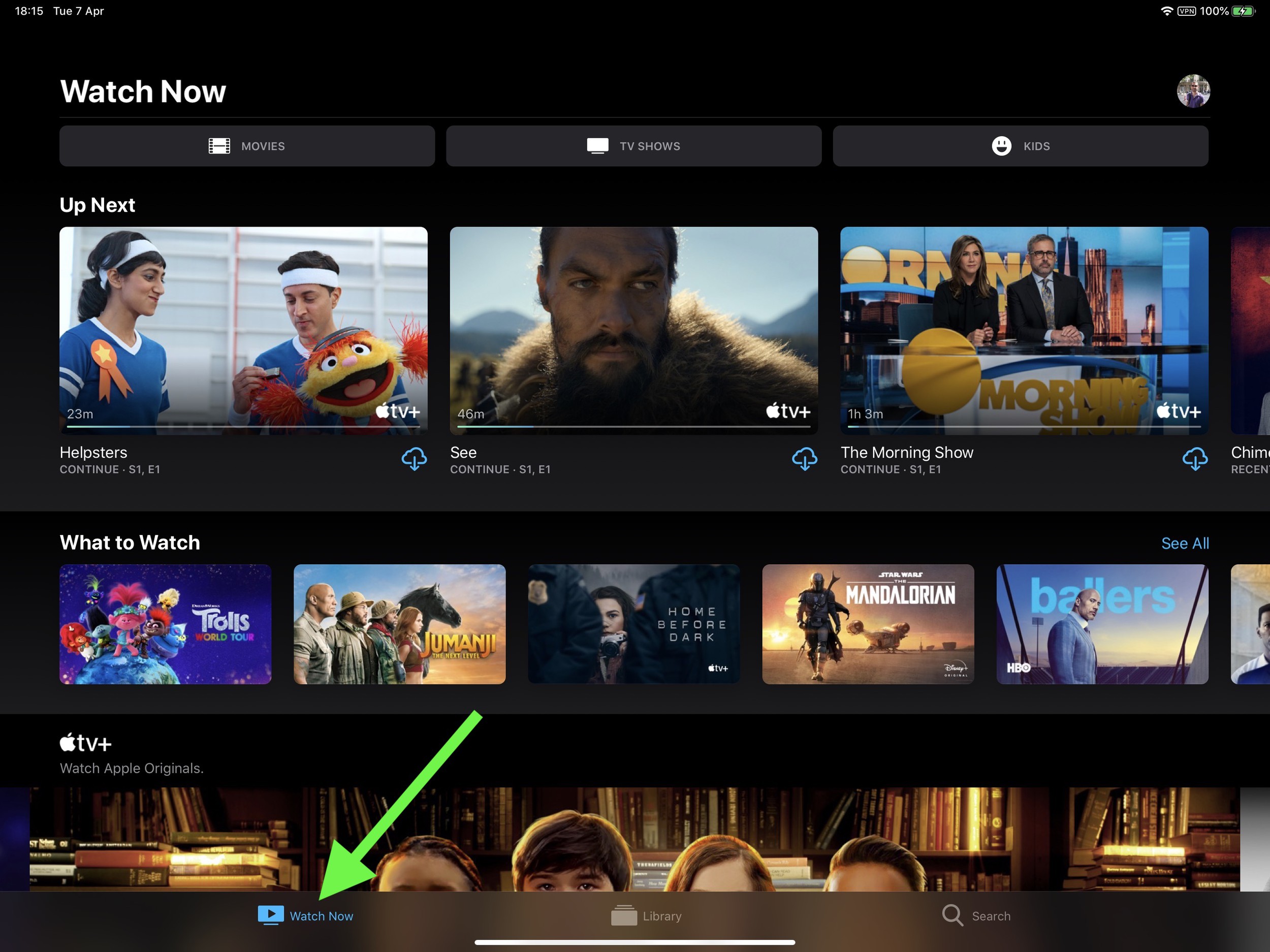This image showcases a web page on a smartphone with a black background, dedicated to viewing options on Apple TV Plus. In the top left corner, very fine text displays the date and time as 18:15 on Tuesday, April 7th. The top right corner shows a fully charged battery icon at 100%. Below this, on the left side, "Watch Now" is written in prominent white text.

Further down, three categories—Movies, TV Shows, and Kids—are listed in white within dark gray boxes. Beneath these categories, "Up Next" in white text indicates the continuing content list. Three rectangular images with rounded corners represent different shows: "Helpsters," "Sea," and "The Morning Show."

Continuing down, the "What to Watch" section offers several options in individual rectangles, including "Trolls," "Jumanji," "Home Before Dark," "The Mandalorian," and "Ballers." Near the bottom of the screen, the iconic Apple logo and "TV Plus" in white text are displayed prominently.

At the far bottom of the screen, a vivid neon green arrow points to the words "Watch Now," located on the left, and next to this are the options "Library" and "Search."